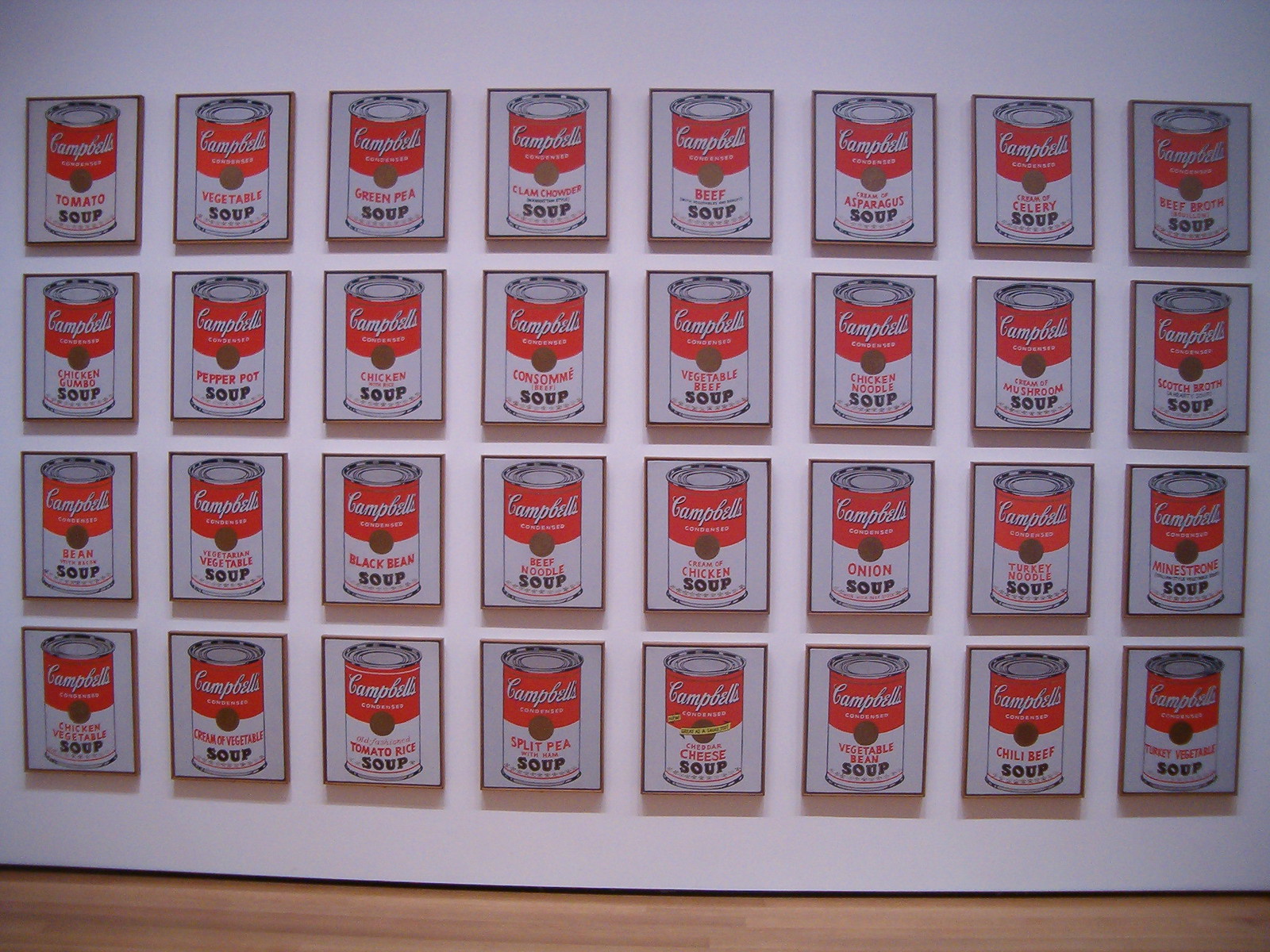This image captures a detailed view of an art installation, likely by Andy Warhol, displayed on a white drywall. The installation consists of a 4 by 8 grid of framed Campbell's Soup can paintings. Each frame casts a shadow on the white wall, and the entire setup hangs above a hardwood or plank floor. The classic Campbell's Soup can design features a red upper half with the Campbell's logo and a white lower half indicating the variety of soup. Although the images initially appear identical, a closer inspection reveals subtle differences in the labels. The types of soup depicted include tomato, vegetable, green pea, clam chowder, beef, asparagus, celery, beef broth, chicken gumbo, black bean, beef noodle, consomme, vegetable beef, and many others. Each frame features a distinct soup variety, showcasing the diverse range of Campbell's Soup products, arranged evenly across the grid on the white gallery wall.